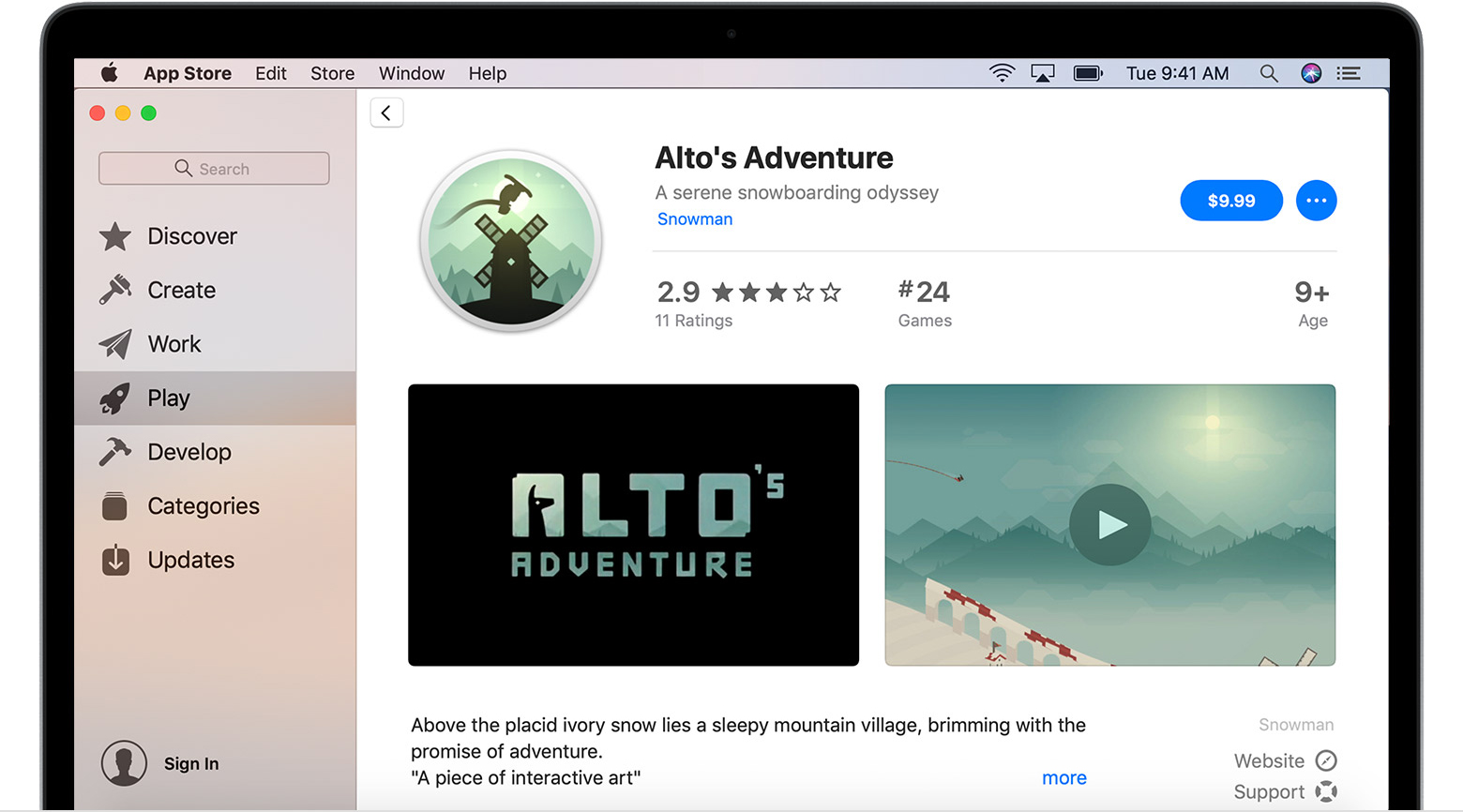The screenshot captures a webpage from the Apple App Store, as evident by the familiar Apple interface and icons. The image appears to be taken on a laptop, given the visible edges of the device at the top and side. 

At the very top of the screen, typical menu options like "App Store," "Edit," "Store," "Window," and "Help" are listed along the menu bar. On the right side of this bar, the status icons display a Wi-Fi signal, what seems to be a square with a rectangular shape and an arrow pointing upwards (possibly representing notifications or downloads), a battery indicator, the time "Tuesday, 9:41 AM," and a magnifying glass symbol for search functionality.

On the left-hand side of the webpage, there's a vertical menu with various categories. This menu is marked by three circle icons, with the first one being red, the middle yellow, and the last one green, likely representing window management buttons (close, minimize, maximize). Below these icons, there’s a search bar followed by menu items labeled "Discover," "Create," "Work," "Play," "Develop," "Categories," and "Updates." The "Play" option is highlighted, suggesting it is the current selection.

The main content area features an app named "Alto's Adventure," described as "a serene snowboarding odyssey." Directly beneath this description is an image of a snowman accompanied by some text in blue. The app's pricing is listed as "$9.99," alongside a button represented by a circle with three white dots. The app has a rating of "2.9 stars" with "11 ratings." It is also noted to be the "number 24 game" in its category and suitable for users "9+." The title "Alto's Adventure" is displayed again on a black background with green text. At the bottom of the section, there is a video preview of the app.